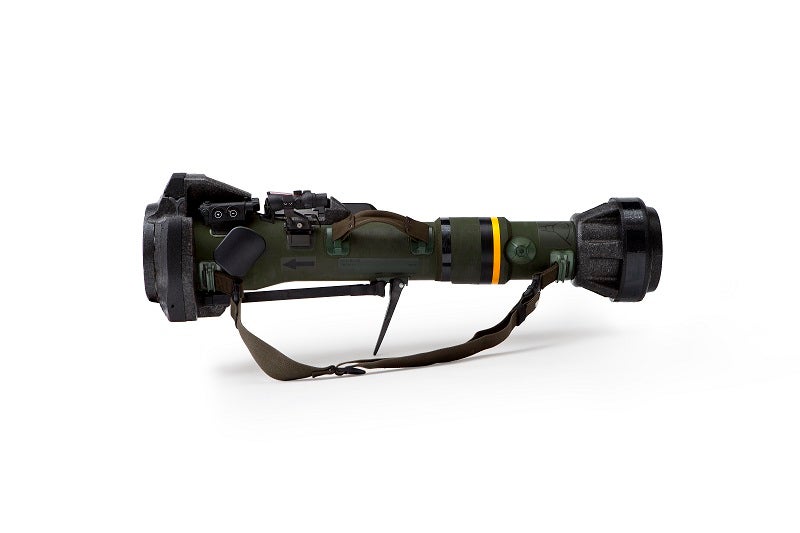Set against a clean white backdrop, the image features a dark green piece of equipment that bears a resemblance to a telescope, magnifying device, or possibly even a weapon such as a scope or a rocket launcher. The object is detailed with a bright gold band situated toward the back and two black knobs on either end. It is equipped with multiple gauges, dials, and buttons, prominently placed on the top and back part of the device. The instrument has a hanging strap, which is dark gray and appears to be sitting on a flat surface, and a smaller brown strap attached to the top that functions as a handle. On the right side of the device, there is a round cap-like end, possibly a lens cover, mirrored by a similar feature on the left side. Additionally, there is a thin, stand-foot style piece at the center bottom of the equipment, designed for balance. This detailed visualization suggests that the object could be military-related.